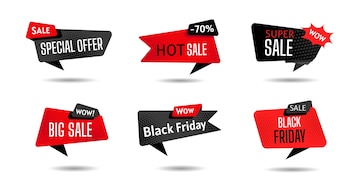This image displays six distinct sale advertisement signs, each with unique designs but a common promotional theme. 

1. The upper left sign features a speech bubble proclaiming "Special Offer" in white text on a grayish-black background, with a red "Sale" tag in the upper left corner.
   
2. Next to it, the top middle sign announces a "Hot Sale" with the word "Hot" in black and "Sale" in white, against a red background. It prominently displays "-70% off" in white text in the upper right corner.

3. The upper right sign reads "Super Sale," where "Super" is in red and "Sale" is in white, set against a black background. A red chat bubble in the upper right corner adds emphasis with the word "Wow."

4. The lower left sign simply states "Big Sale" in white text on a red background. It also features a "Wow" bubble in the upper right, styled in white text on a black background.

5. The middle bottom sign is dedicated to "Black Friday," written in white text on a black background. The word "Wow" appears again in the upper right corner, this time in white text on a red background.

6. The lower right sign is another "Black Friday" promotion, showcasing white and black text on a red background. It includes a black speech bubble with the word "Sale" in white text in the upper right corner.

The consistent use of vibrant colors like red, white, and black, along with attention-grabbing phrases like "Special Offer," "Hot Sale," "Super Sale," "Big Sale," and "Black Friday," ties these advertisements together, emphasizing urgency and significant discounts.